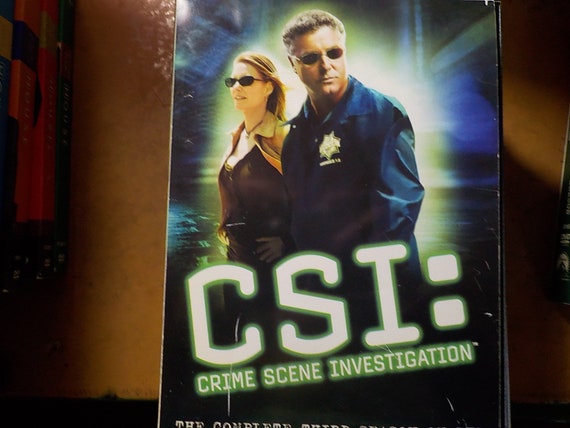The close-up image focuses on a vintage-looking DVD box set for the television show "CSI: Crime Scene Investigation," prominently featuring the title in large white letters outlined in green. The DVD case has a blue background with a distinctive green spotlight. Within this spotlight stand two main characters from the show: a middle-aged, gray-haired man wearing small, oval sunglasses and a blue jacket adorned with an insignia that appears to be a star, and a woman with reddish-blonde, tied-back hair, also wearing sunglasses and a brown shirt. They are both staring intently, with the man looking directly at the camera and the woman standing behind him, glancing off to the side. The words "The Complete Third Season" are visible but partly cut off at the bottom. The DVD case is placed on a wooden table, and the overall aesthetic of the box set and table gives the image a nostalgic, slightly worn feel.